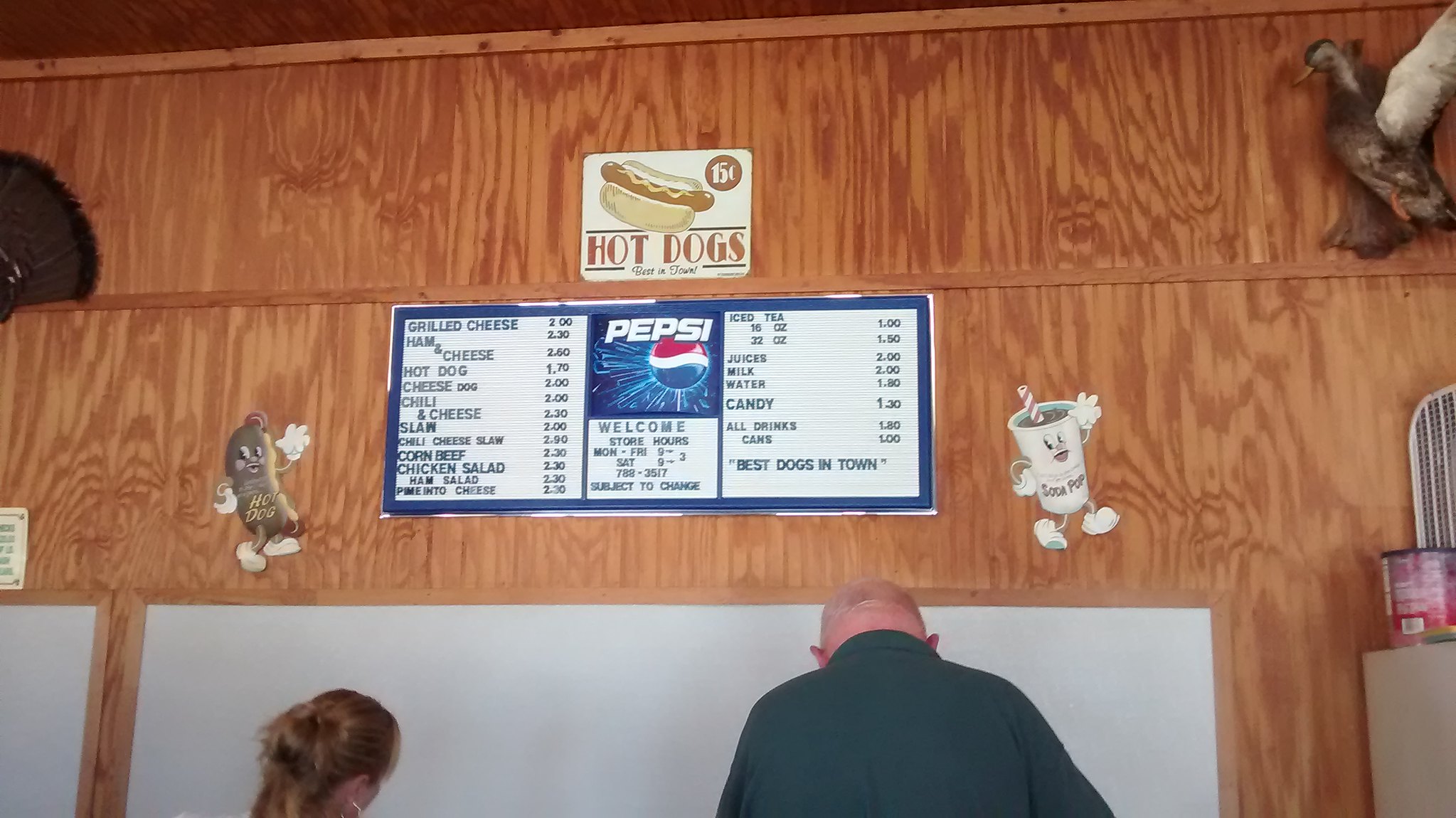In this photograph taken inside a classic diner-style restaurant, the camera angle is directed upwards towards the upper part of a wall adorned with vibrant signage. Prominently featured is a colorful sign advertising "Hot Dogs," complete with an illustrated hot dog that connotes the establishment's signature item. Below this inviting sign, a vintage Pepsi-Cola branded menu board lists a variety of comfort foods: grilled cheese, ham and cheese sandwiches, hot dogs, cheese dogs, slaw, and corned beef. On the right side of the menu board, the drink options are displayed, including ice teas, juices, and bottled waters. There's even a selection of candies available for a sweet treat.

Beneath the menu, two patrons are seen from behind, subtly contributing to the scene without distracting from the primary focus of the image. One is a woman, her back and hair visible to the viewer. To her right stands an older man, his dark green polo shirt and thinning, gray hair suggesting his advanced age. The detailed composition of the photograph captures the nostalgic charm and welcoming atmosphere of a traditional American diner.